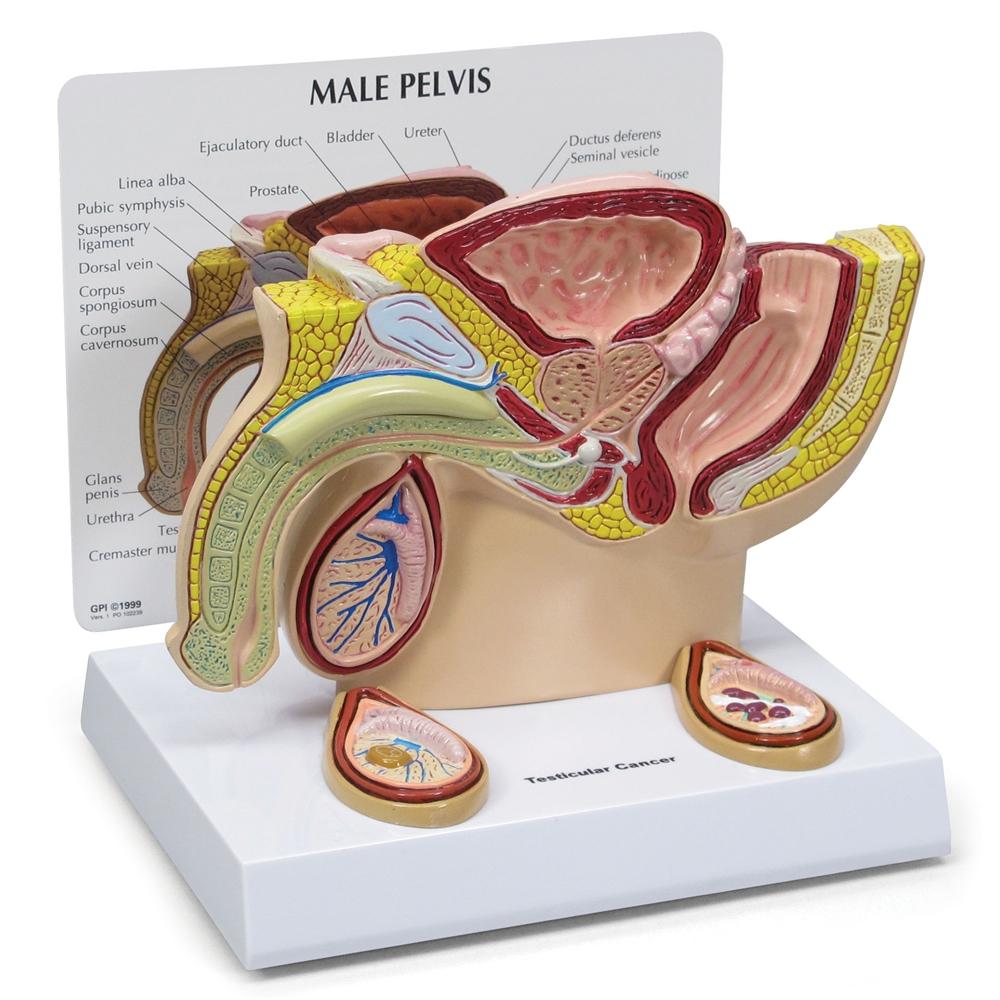**A highly detailed educational display of the male pelvic region stands prominently on a white platform. At the forefront, a meticulously crafted 3D plastic model illustrates the intricate anatomy, including the prostate, bladder, ureter, and other male reproductive organs. Each component is vividly colored in shades of yellow, burgundy, light pink, blue, white, and gray to enhance clarity. Behind this 3D model, a white card with black font reads "Male Pelvis" and provides detailed annotations of the various parts. The card also features a matching printed diagram that reinforces the information presented by the model. Additionally, a section of the display is labeled with "Testicular Cancer," emphasizing its educational purpose. This comprehensive visual aid is reminiscent of the type of detailed anatomical models often found in a doctor's office.**